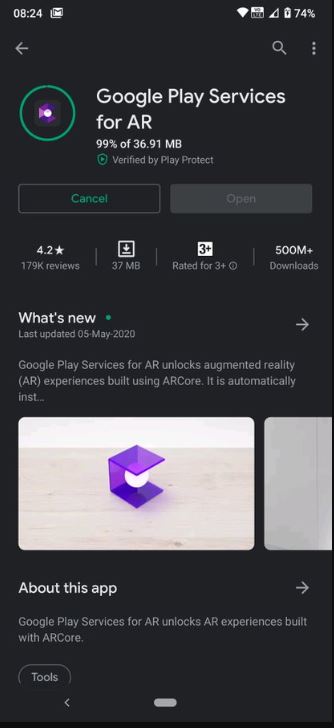In this image, we see a detailed screenshot of a cell phone displaying a page from an app. At the very top is the phone status bar which includes, from left to right, a clock, an email notification icon, a Wi-Fi signal indicator, a network strength meter, and a battery level icon.

Below the status bar, the prominent section of the screen features a black background. At the very top of this section is a search icon. Just beneath this icon, in white font, it reads "Google Play Services for AR". Directly under this text, it states "99% of 36.91 MB, verified by Play Protect."

Following this information are two buttons labeled "Cancel" and "Open".

Further down, we encounter sections dedicated to user reviews, download size, rating, and the number of downloads. An informative segment labeled "What's New" reveals that the last update was on 5th May 2020. The description notes, “Google Play Services for AR unlocks augmented reality experiences built using ARCore. It is automatically...,” but the text is cut off and incomplete.

Lastly, there's an image of the logo for Google Play Services for AR, depicted as a purple box encasing a white ball.